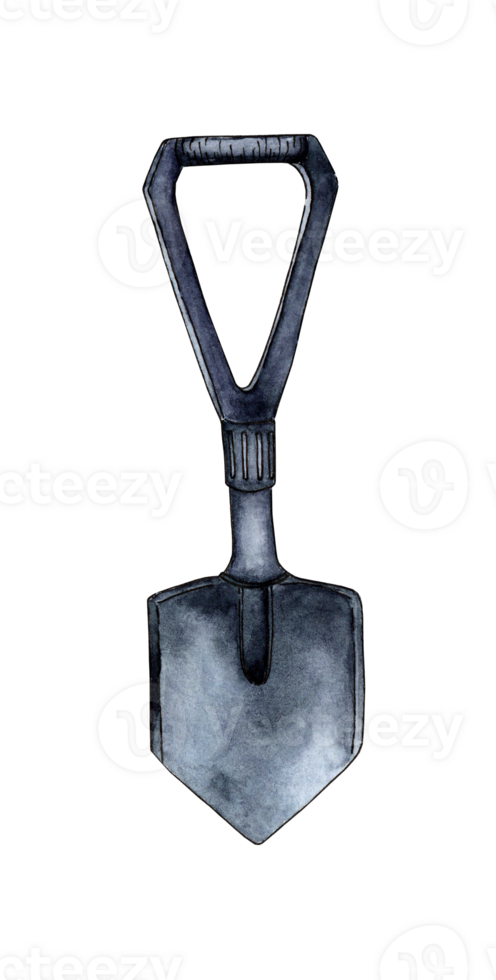The image depicts a gardening spade with a distinctive, ergonomic design, prominently featured against a stark white background. The spade, which appears to be a hand-drawn rendering rather than an actual photograph, is detailed and realistic, almost resembling watercolor and ink artwork. The spade itself has a pointed blade at the bottom and an exceptionally short neck or stem, approximately the same size as the blade, with an adjustable knob possibly suggesting some adjustability. The handle above is notably large, triangular-shaped, and has an open middle, allowing for a firm grip. The entire tool is shaded in dark grey tones, conveying an aged appearance. Across the image, there is a watermark with the text "Fizzizi" encircling a V-shape symbol, and another watermark labeled "O-T-Z," indicating its source as an online platform likely selling or showcasing this spade as part of a stock image collection.